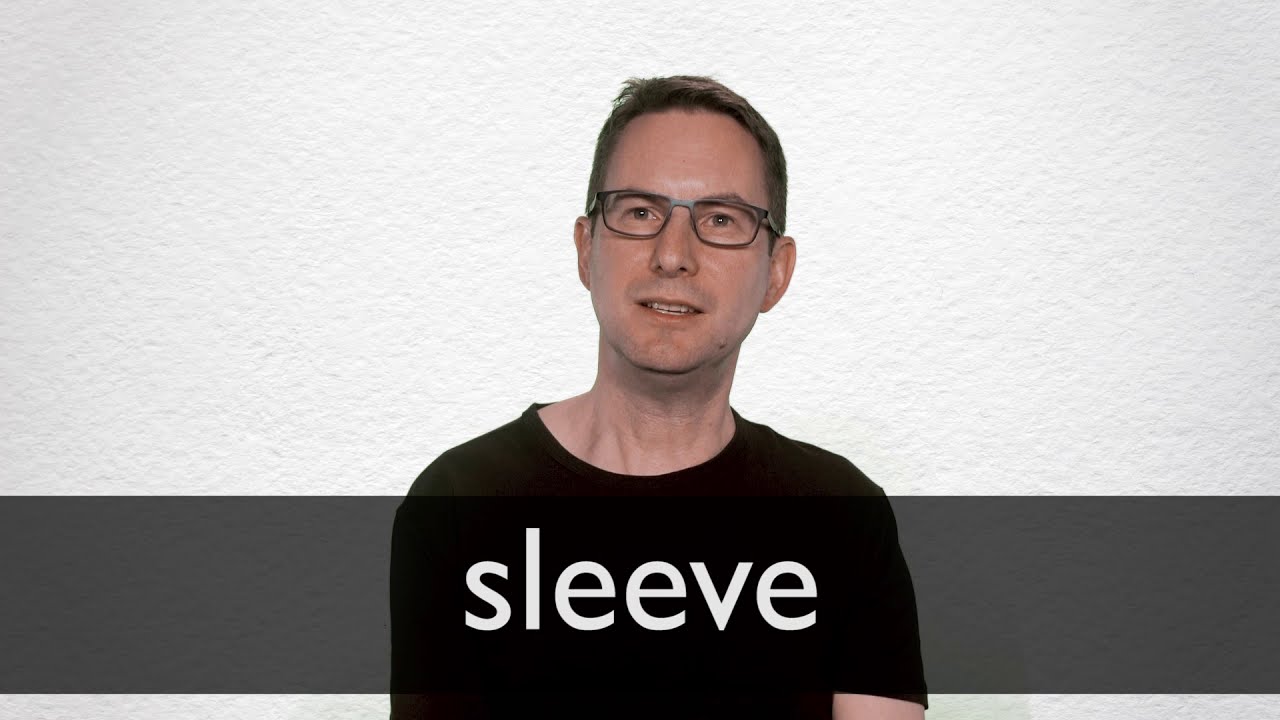The image features a Caucasian man who appears to be in his 30s, wearing prescription glasses with very clear lenses through which his brown eyes are visible. He has short, dark brown hair that is closely cropped to his head. His complexion is fair, and he appears clean-shaven, although there might be a faint hint of a mustache that's either just starting to grow back or not fully filled in. 

His mouth is slightly open, showing both the top and a bit of the bottom ridge of his teeth, as if he is in the process of speaking. He is wearing a black t-shirt with the word "sleeve" written in all lowercase letters across the chest, stretching from one shoulder to the other. The background comprises a textured white wall with a smooth gray horizontal stripe running underneath it. The overall setting puts the focus on the man, who seems to be looking past the camera at something in the distance. 

There is also a semi-transparent black bar at the bottom of the image, displaying the word "SLEEVE" in large, white text, suggesting that this could be a thumbnail or still from a video. The image captures a small reflection on his forehead and dots of reflection in his eyes, highlighting the intricate details of the scene.